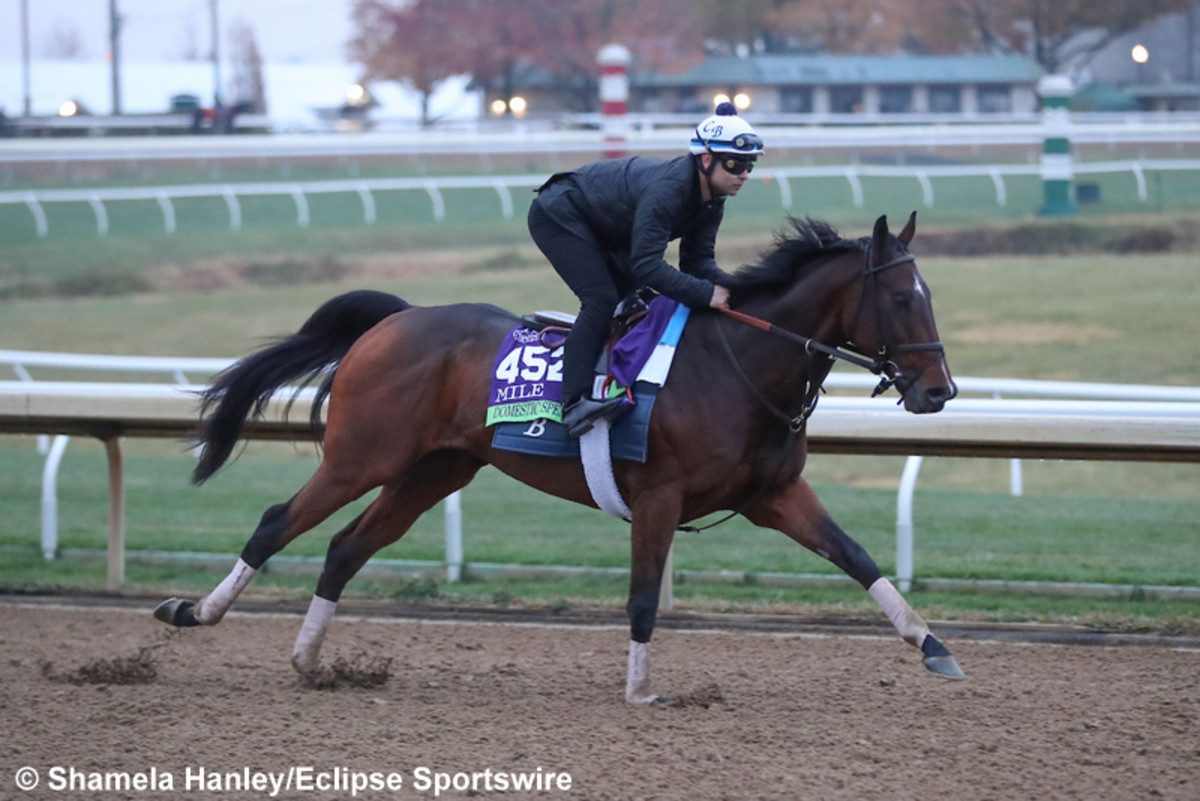In this photograph, a dynamic scene unfolds of a horse race in progress, captured with striking detail. At the forefront, a magnificent racehorse, exhibiting a rich dark brown to black coat with distinctive white socks, gallops powerfully along a racetrack. The horse's black mane and tail flutter dramatically with its movement, accentuating its robust form. Draped over the horse is a purple blanket adorned with the number "452 mile" in white writing, layered atop another green and blue cloth with additional text, though it's partially obscured.

Astride the horse, the jockey is poised with athletic precision, crouching over the horse rather than sitting fully in the saddle, enhancing the sense of speed and agility. The jockey dons a striking all-blue outfit, complete with blue shoes, a navy blue suit, and a blue and white helmet featuring the letters "C B" and topped with a blue pom-pom. The jockey also wears protective glasses, adding to the air of professionalism and preparedness.

The image is framed with a copyright notice in the bottom left corner naming Shyamala Hanley of Eclipse Sportswire, a detail that authenticates the photograph and underscores its professional capture. In the background, slightly out of focus, a building and tall cones, one red and white, the other green and white, outline the scene, accompanied by trees that hint at the presence of water behind them. A light blue sky spans the top of the image, transitioning to darker tones interspersed with red and green leaves, adding depth and context to this vivid portrayal of equestrian sport.